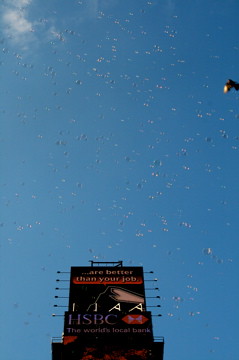The photograph captures an upward perspective of a cityscape, dominated by the sky which is a light blue hue with patches of white clouds gathered in the top left corner. The image is rectangular, with the left and right sides extending longer than the top and bottom edges. The sky is whimsically filled with innumerable soap bubbles that span across the entire frame, adding a magical touch to the scene. 

Situated prominently in the bottom center of the image is the roof of a building adorned with two rectangular billboards. The lower billboard is black featuring bold white text that reads, "HSBC, the world's local bank." Positioned directly above it, the second billboard portrays a mountain landscape on its bottom half, accompanied by a provocative message in white text at the top stating, "Are better than your job." Together, these elements create a captivating and thought-provoking visual narrative that invites viewers to ponder the juxtaposition of corporate messaging and the allure of nature amidst a whimsical bubble-filled sky.